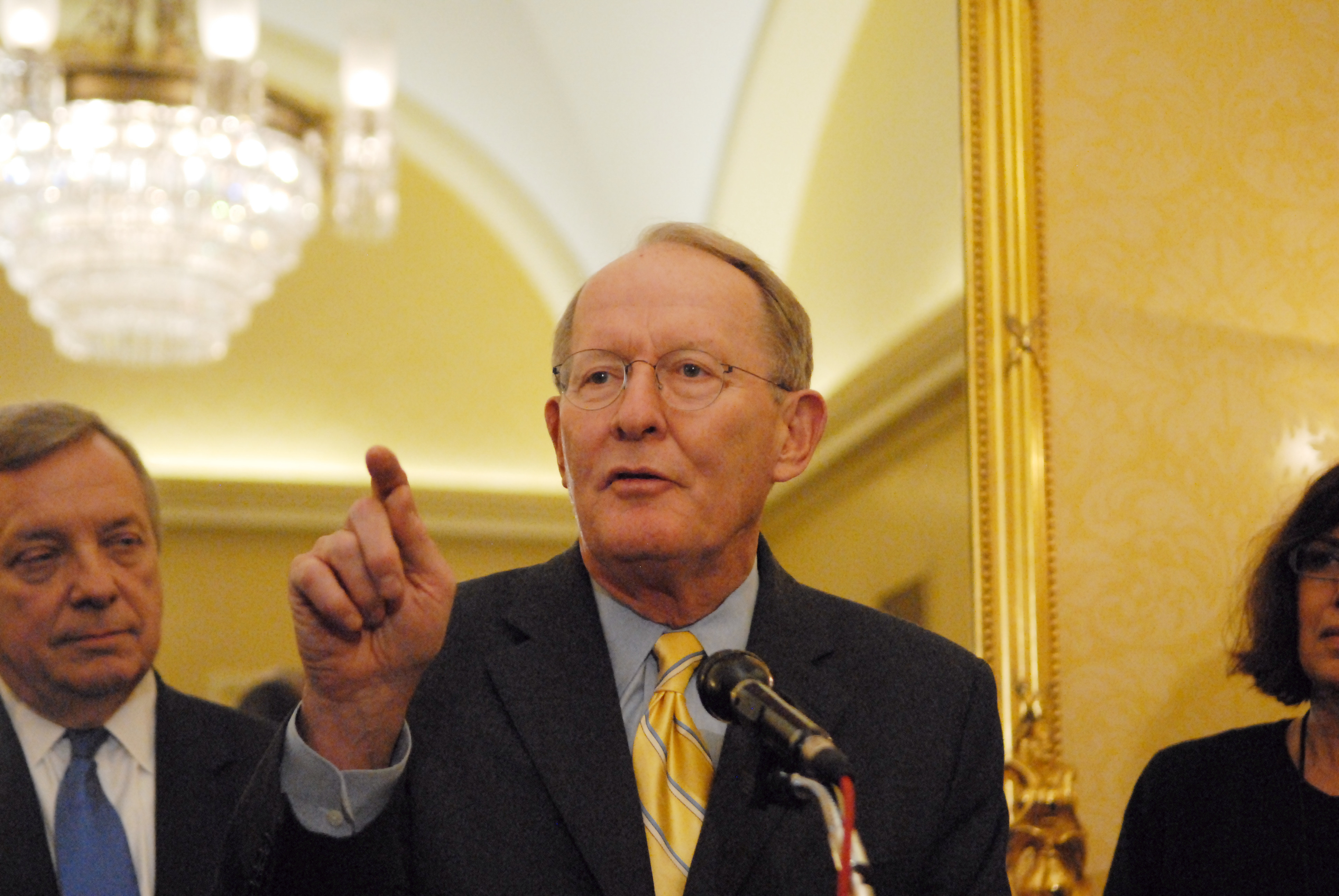In the close-up photograph, we see a very old and wrinkly politician, possibly Senator Lamar Alexander, who is dressed in a dark blue suit with a light blue shirt underneath and a yellow necktie adorned with blue and white stripes. He sports thin, clear glasses and short, receding blonde hair, giving him a distinguished yet aged appearance. Holding a black-wired microphone with a red wire on a stand, he is captured mid-speech with his right hand raised, pointing towards something or someone in the crowd to our left. Beside him on our left, his right, stands another elderly gentleman with gray hair, wearing a white shirt, a blue tie, and a suit jacket, intently observing the speaker. In the background, on the speaker's left, our right, is a woman with dark, short hair and glasses, partially obscured, wearing a black shirt. The photo is set in a bright, opulent ballroom, marked by a grand chandelier in the top left corner and golden mirror edges on the walls, enhancing the formal atmosphere of the scene.